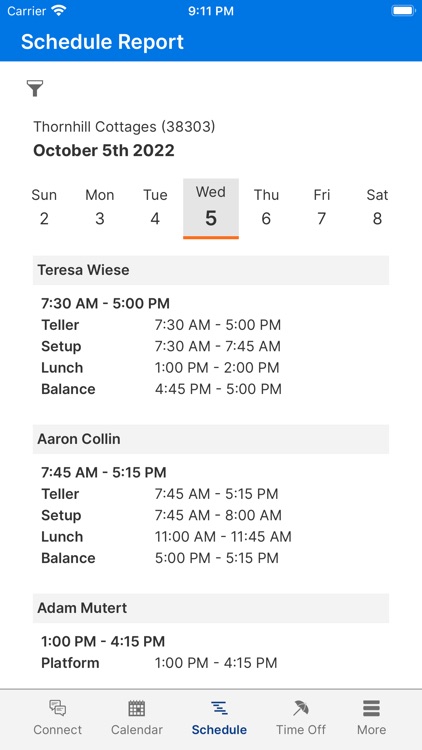This is a detailed screenshot of a schedule report viewed on a mobile device. At the very top, the title bar reads "Schedule Report" in white text. Below the title bar, the header displays the name "Thornhill Cottages (38303)" and the date "October 5th, 2022" in bold, black text.

The calendar section underneath outlines the days of the week with specific dates: Sunday (2nd), Monday (3rd), Tuesday (5th), Thursday (6th), Friday (7th), and Saturday (8th). The image is divided into three sections, each listing three contacts associated with specific shifts.

The first section indicates the position of President, currently held by Teresa Weiss. The subsequent sections list individuals named Collin, Mandy, and Greg (identified as the speaker's great-grandfather) assigned to their respective shifts for day work. This detailed schedule provides a clear overview of the assigned personnel and their respective workdays.